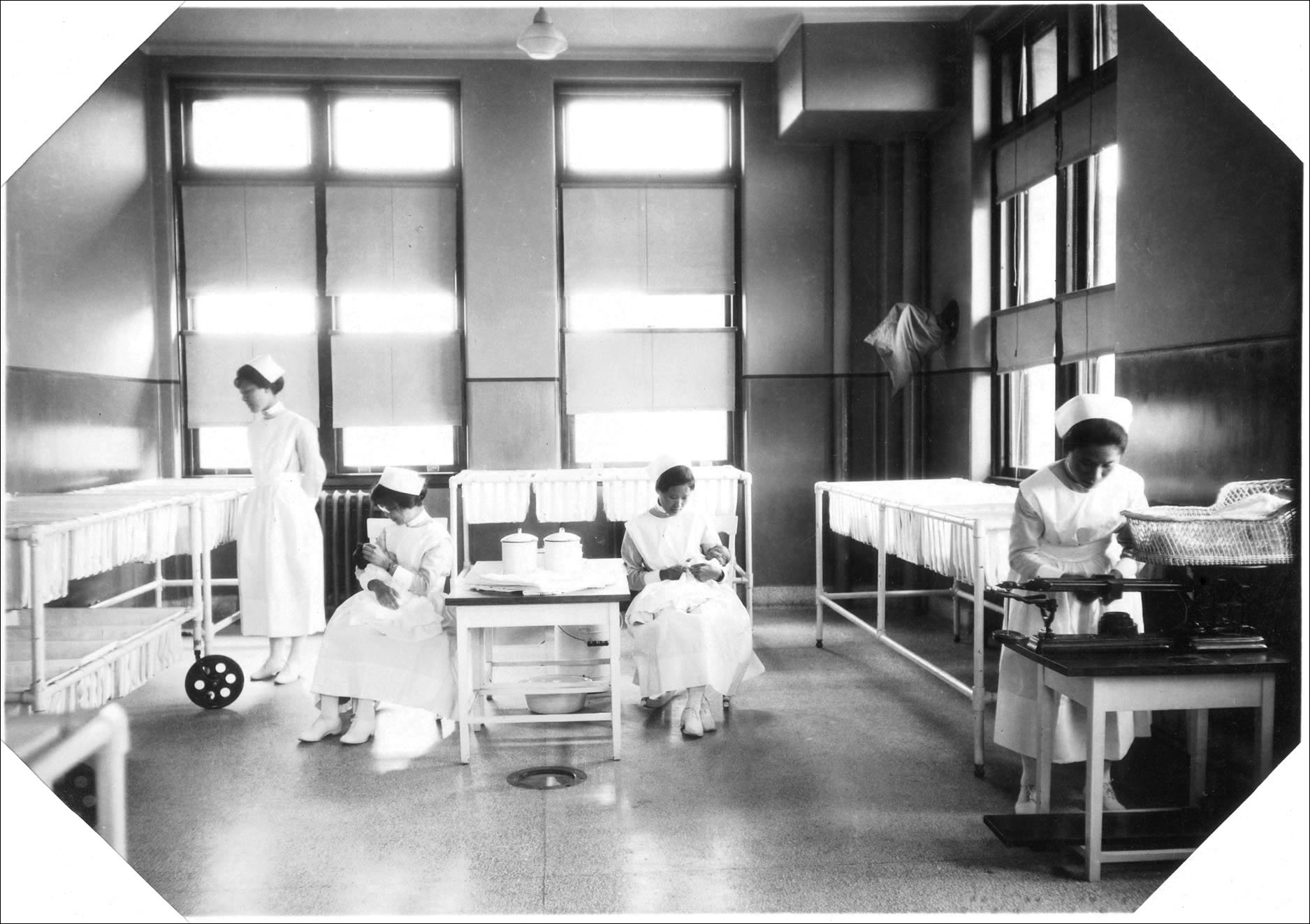This is a black-and-white photocopy of an old hospital nursery, possibly from the Edwardian period. The clean and well-lit room, with its shiny floors and numerous windows, is occupied by four nurses wearing classic white uniforms, including long-sleeve dresses, full-length aprons, caps, stockings, and shoes. Two of the nurses are seated, each cradling and feeding a newborn baby wrapped in a blanket. The nurse on the left is looking over at baby cradles arranged on racks, while the nurse on the right is bent over a table, possibly weighing a baby in a bassinet. In the background, a small table with several pots is visible, adding to the methodical arrangement of the room. The photo has cut-off corners, adding to its vintage charm and historical significance.